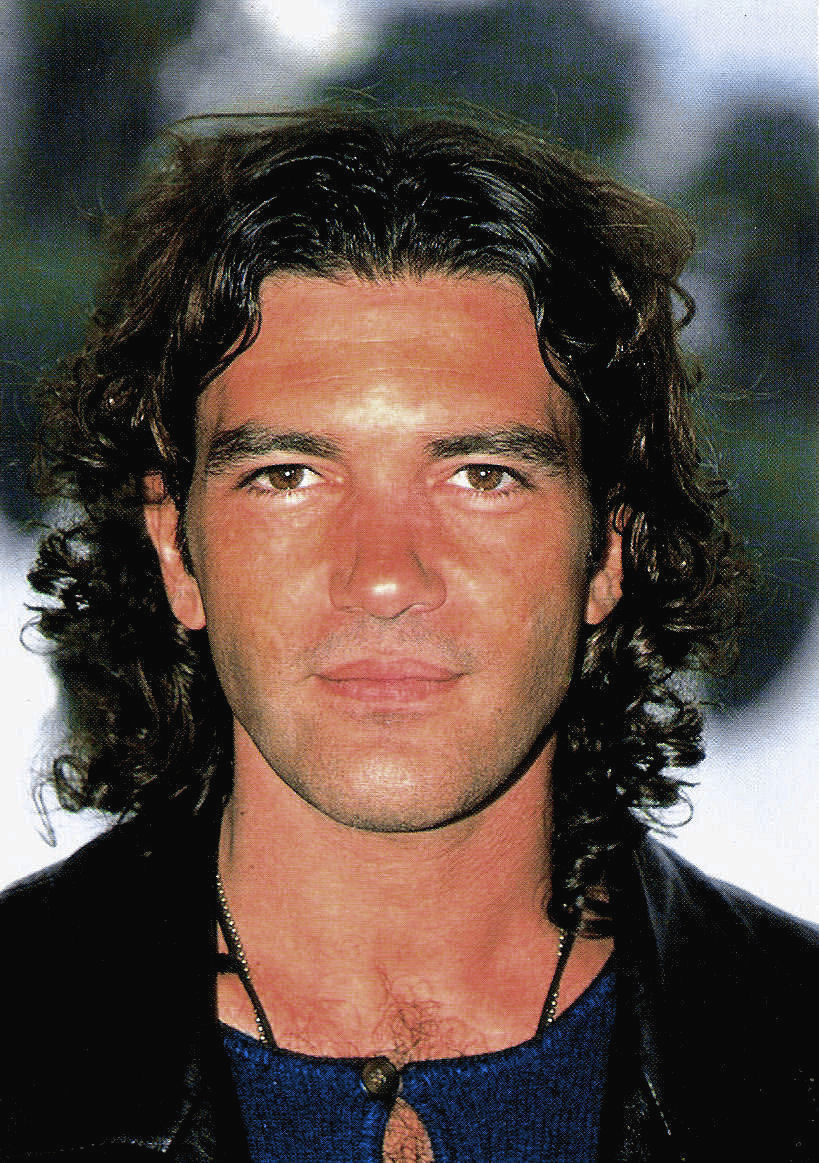This portrait-oriented photograph, likely taken outdoors during the daytime, features a man who bears a resemblance to Antonio Banderas from the 1990s. He appears to be in his 30s with medium-length, curly black hair that reaches just above his shoulders. His skin has a light brown tone with a reddish hue, suggesting he might be tanned or slightly sunburned. The man has a strong facial structure, accented by thick black eyebrows and medium brown eyes, which are open and directed slightly off to the side, giving him a thoughtful yet neutral expression. His slightly unshaven look features a noticeable five o'clock shadow. He is dressed in a blue shirt that buttons at the collarbone, partially revealing a hint of chest hair, and he layered it with a black jacket. A faint glimpse of a necklace can be seen peeking out from under his shirt. The background is blurred, displaying an indistinct blend of white and green, possibly indicating some greenery, which places the focus squarely on him.